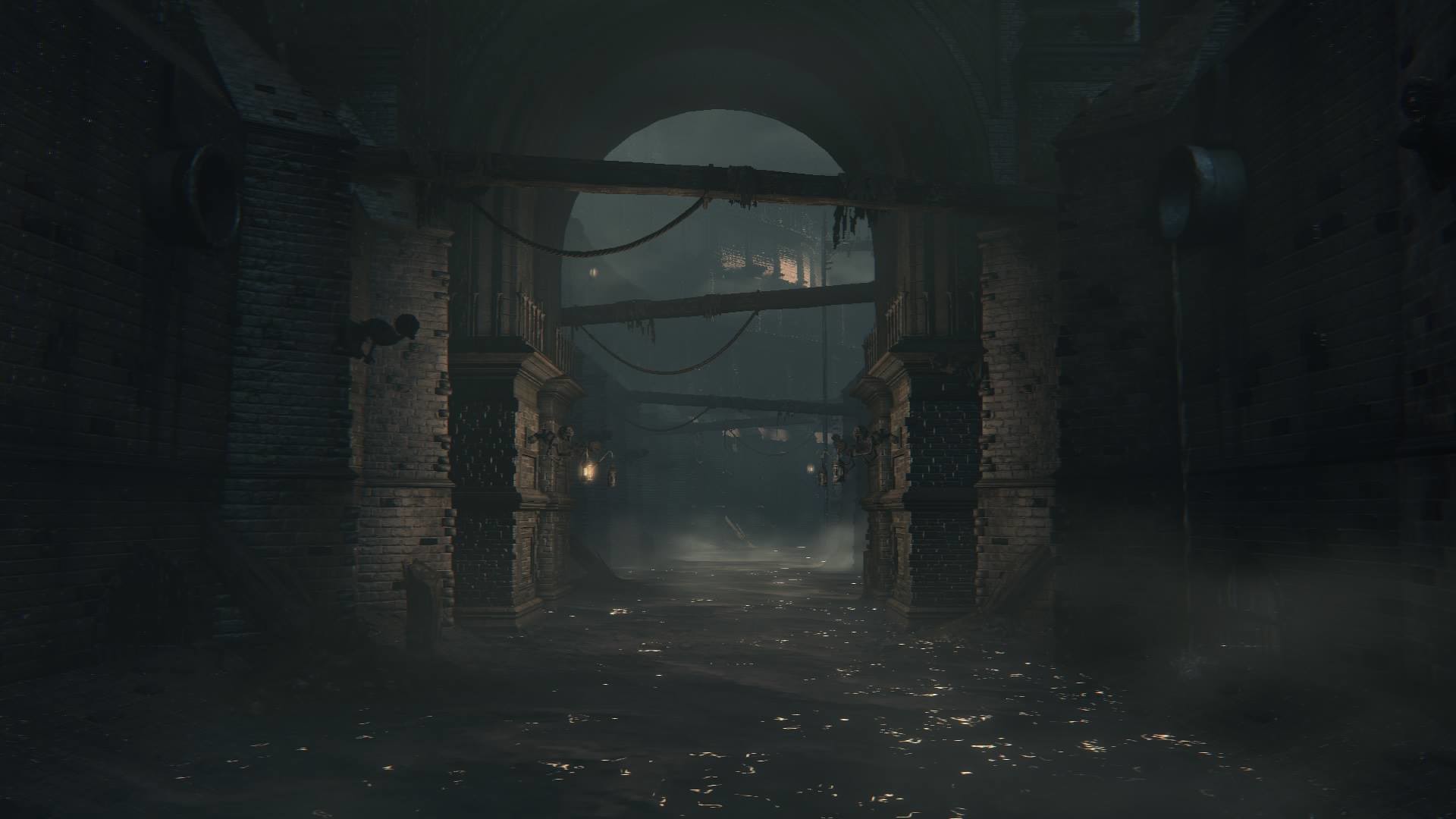In this image, we are presented with a dimly lit, eerie setting within a video game that depicts the interior of an old, abandoned building. The image is in landscape orientation and shows a gloomy hallway or alleyway within a medieval or 1800s-style structure. The scene is characterized by dark, crumbling brick walls that are light-colored, possibly white or gray and a floor that appears black and littered with debris. Along the floor, there are gray and white speckles, giving the impression of either ground or water.

On either side of the image, two dark gray columns are visible, and above, the ceiling is held up by exposed, rusting iron beams or pipes. These girders support the exterior walls of the building. In the center of the image, there is a keyhole-shaped archway comprised of brick, through which one can see an ominous, dark area beyond. This area outside the archway might be an open courtyard or a dark, smoggy exterior space with faint lights and windows visible in the distance.

Adding to the haunting atmosphere, there appears to be a streetlamp or lantern situated at the bottom left of the archway. The overall ambiance is one of gloom and eeriness, accentuated by an emerging fog rising off the ground, evoking the feeling of a dark alleyway where one would not want to be caught, whether during the day or night. The scene effectively conveys a sense of desolation and mystery, typical of an old, ruined building in a forsaken part of town.